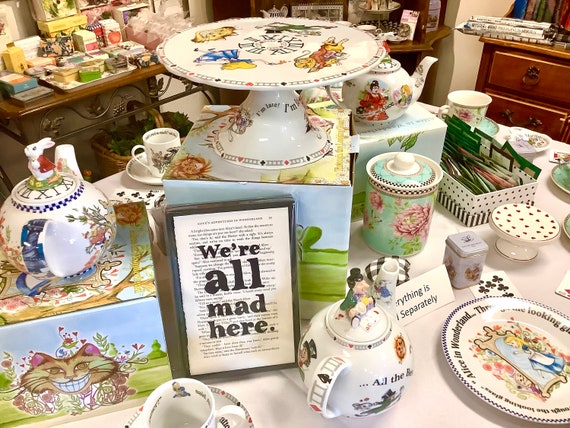The image depicts a charming and whimsical display likely situated in an antique store or themed shop, evocative of the Mad Hatter's Tea Party from "Alice in Wonderland." The centerpiece is a white table adorned with an array of intricately decorated teapots, china, and plateware, many featuring cartoon imagery. A framed piece of paper in the center bears the quote "We're all mad here," reinforcing the Alice in Wonderland theme. Notably, there are various teapots, one of which has a Mad Hatter figure, complete with a top hat, as its lid, and another adorned with a standing rabbit, possibly referencing Peter Rabbit. Complementing the teapots is a white, ornamented china cake stand, wrapped with slightly obscured cartoon decorations, positioned on a box. 

The table also holds a metal tin without a lid, filled with teabags of different shapes and sizes. Encircling this setup, the background reveals armoires and old wooden furniture, brimming with assorted trinkets. Among these details, several white plates showcase different "Alice in Wonderland" characters, further enhancing the fantastical theme. The entire scene is a delightful assemblage of vintage charm and storybook nostalgia.